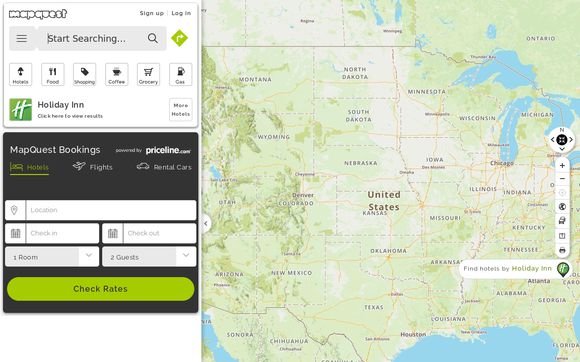This detailed caption illustrates a cropped screenshot of the MapQuest travel section, composed of multiple distinct elements arranged in an organized layout. On the left side, there are two smaller boxes stacked vertically; the top box is predominantly white, featuring the MapQuest logo in black at the top left corner and a prompt to "Sign Up or Log In" displayed in small black letters at the top right. Beneath this, a gray menu box is situated to the left, adjacent to a larger text box on the right that encourages users to "Start Searching" accompanied by a magnifying glass icon on the far right. Just beside this, there is a green arrow button directed leftwards. 

Below this setup, six small category boxes are presented in a grid, each containing an icon at the top and a descriptive name at the bottom. Underneath these categories, an advertisement for Holiday Inn is placed, inviting users to "Click Here" and explore more hotel options. The second smaller box on this left section has a black background and is dedicated to MapQuest bookings, indicated at the top left corner, and is powered by Priceline.com as noted on the right side. This box categorizes options for hotels, flights, and rental cars, each accompanied by respective text boxes for user input. At the very bottom of this box, a prominent green button labeled "Check Rates" invites users to finalize their searches.

On the right side of the screenshot, a much larger square predominantly displays a map of the United States, providing a visual context for the travel information and tools available within the MapQuest interface.